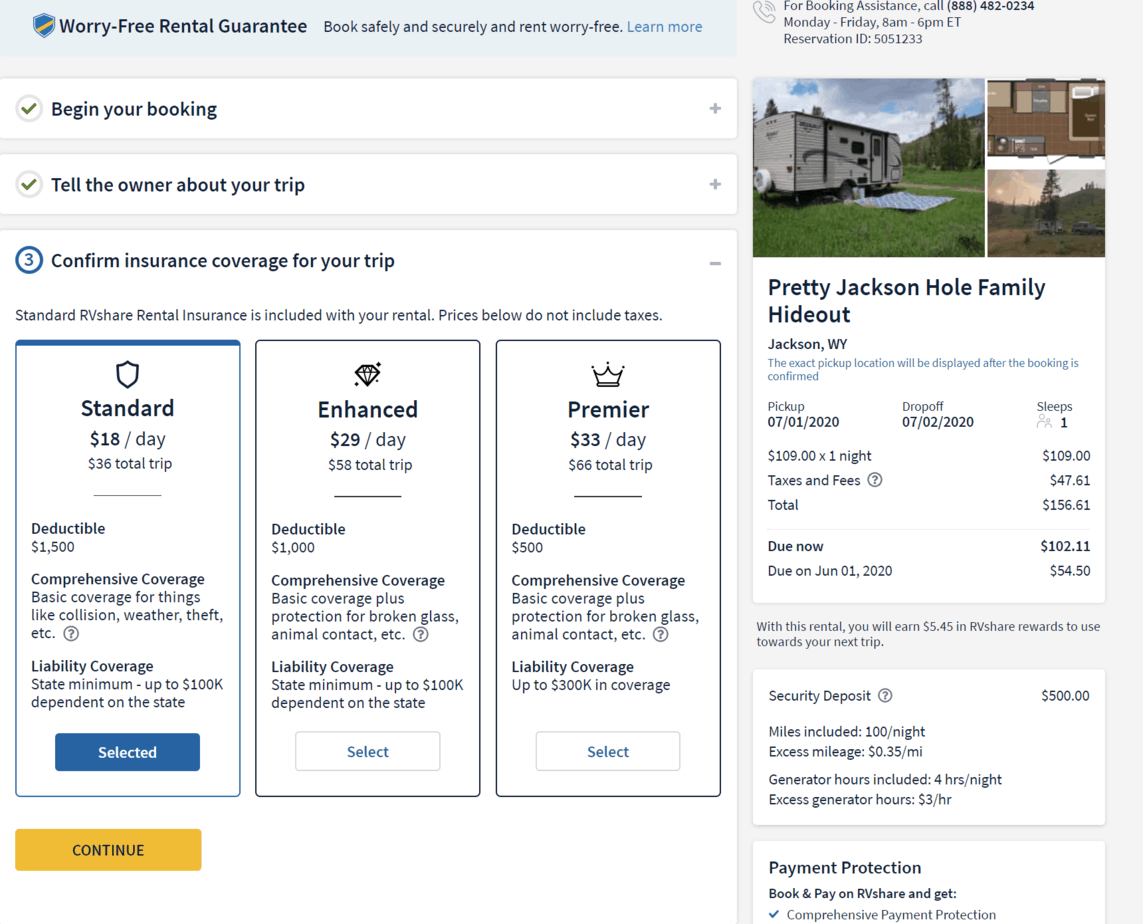This is a detailed screenshot of a computer screen displaying a website for renting holiday accommodation. The interface is shown in landscape mode. 

In the top left corner, there is a blue shield logo with a yellow diagonal line through it, labeled "Worry-Free Rental Guarantee." Below this, text reads, "Book safely and securely and rent worry-free. Learn more." Adjacent to it on the right, there is a message stating, "For booking assistance, call 888-482-0234 Monday to Friday, 8 a.m. to 6 p.m. ET," followed by the reservation ID, "505-1233."

Returning to the left, a drop-down menu titled "Begin your booking" is visible. Below that, another drop-down menu reads, "Tell the owner about your trip." Further down, an open menu labeled "Confirm insurance coverage for your trip" presents three different options: Standard, Enhanced, and Premier, each with varying costs and levels of protection. The "Standard" option is selected by default, while the "Enhanced" and "Premier" options have unselected buttons next to them. A prominent yellow button labeled "Continue" is positioned at the bottom of this section.

On the right side of the screen, there is another menu displaying imagery associated with the rental. The images include a main photo of a caravan situated in a green field with hills in the background, alongside two smaller images – one showing a floor plan and the other depicting the surrounding scenery. Below the images, the listing title "Pretty Jackson Hole Family Hideout - Jackson, WY" is displayed, with a note stating that the exact pickup location will be revealed after booking is confirmed. Additional rental details include pickup and drop-off dates, accommodation for one person, and pricing information, including taxes and totals.

Beneath these details, on a white background, it mentions that the rental includes "$5.45 in RV Share Rewards." Further, within a white square, there is information on the security deposit amount, miles included, excess mileage, generator hours included, and excess generator hours. The text cuts off at the bottom of the screenshot, hinting at information regarding payment protection with a note mentioning, "Book and pay on RV Sharing to get comprehensive payment protection."